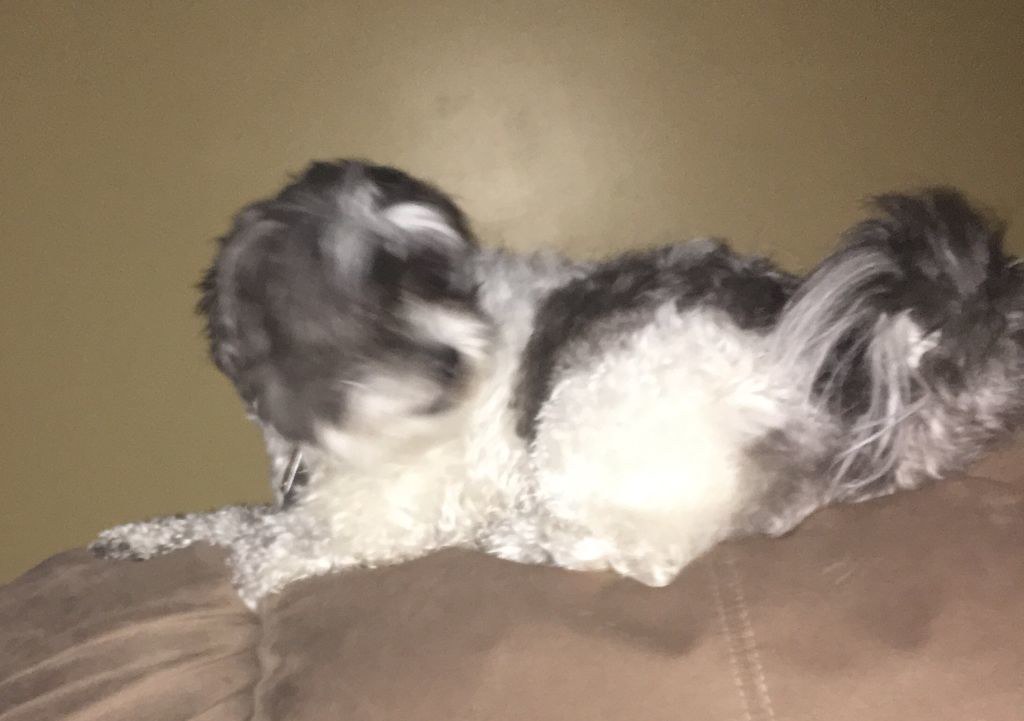In this image, we are looking at a slightly out-of-focus photograph of a dog lying horizontally on a maroon couch. The dog is of small to medium build with fluffy, black, and white fur. Its tail is particularly fluffy, predominantly black and turning white toward the tip. The bottom portion of this dog features white, curly fur which extends to its paws, and as we move upward, the fur transitions to darker hues, culminating in a predominantly black head, which is more out-of-focus than the rest of the image. The dog has its head turned back towards its tail, presenting a restful pose. The background reveals a smooth brown wall that contrasts with the softness of both the dog's fur and the couch fabric.